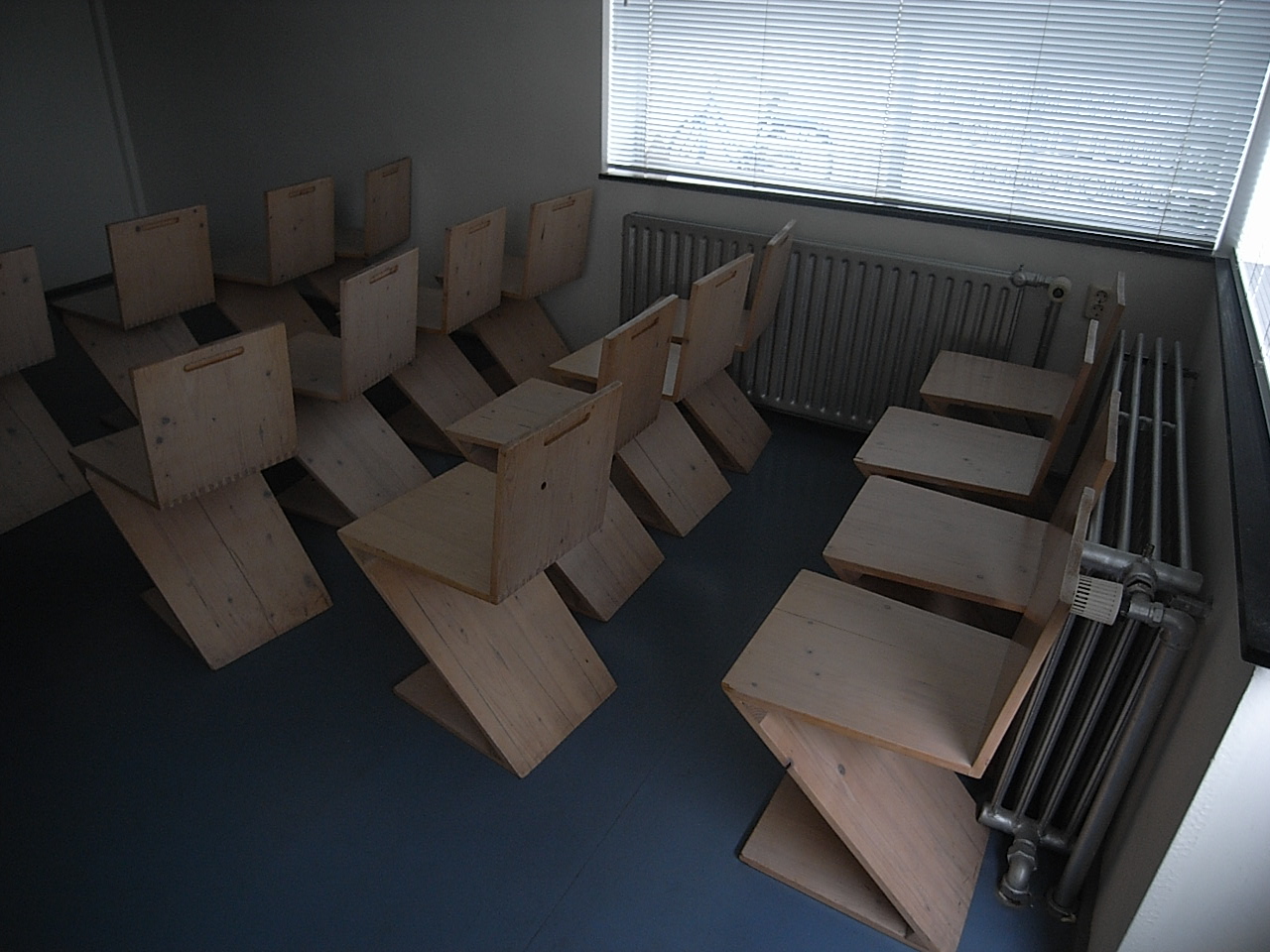The photograph captures a dimly lit, seemingly small room that resembles a classroom, where natural light filters in through windows. The primary source of light comes from a window situated at the top right of the image, featuring horizontal slatted blinds that are mostly closed. Through the slats, a bicycle faintly comes into view, leaning against something outside. Below this window, a hydronic heater stretches along the wall. Additionally, there is another window at the rear of the room accompanied by a similar heater. The floor comprises blueish dark grey carpet tiles, while the walls are off-white. Four rows of modern, uniquely designed wooden chairs furnish the room, each row containing four chairs. These chairs, made from light-colored, smooth, unfinished wood, feature a slightly tilted backrest, a flat seat, and a Z-shaped structure. This design is characterized by a piece of wood extending diagonally from the front of the seat down to the floor, aligning with the back of the chair, with another piece extending forward as a base. All chairs are oriented towards the left corner of the image, enhancing the room’s modern aesthetic amidst its subdued lighting.